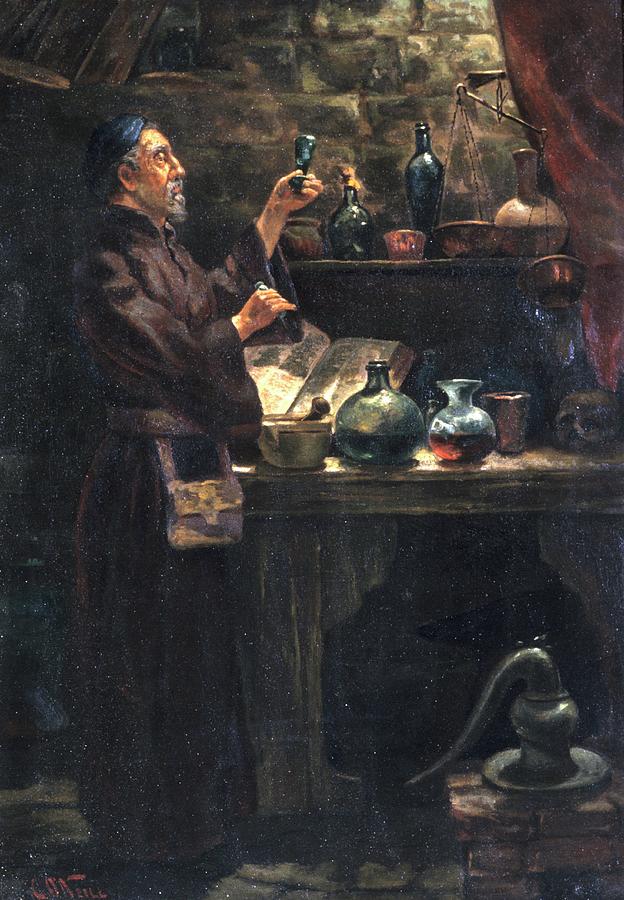This image is a richly detailed, old oil painting depicting a scene reminiscent of the Middle Ages or Biblical times. At its center stands an aged man with gray hair and a matching beard, clad in a long, brown robe with a blue head covering and a satchel around his waist, giving him a monk or preacher-like appearance. The man is engrossed in his work at a cluttered wooden table, situated within a dimly lit, cobblestone walled room that suggests an ancient castle or alchemist's quarters. 

He carefully examines a glass flask held aloft in his left hand, while his right hand holds a mysterious object. Surrounding him on the table are various flasks, vials, and bottles filled with differently colored liquids, indicating his involvement in some chemical or alchemical process. An open book with presumably intricate recipes lies in front of him, alongside a mortar and pestle, hinting that he has been crushing ingredients to concoct potions or tinctures. Additional items like a scale and numerous other containers and tools are strewn around, enhancing the atmosphere of meticulous, scholarly experimentation.